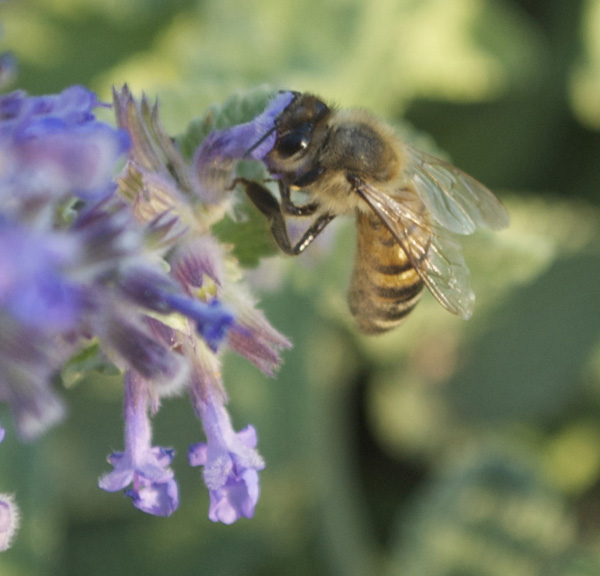This detailed close-up image captures a moment in daylight where a fuzzy bumblebee, characterized by its big black eyes, orange and black-striped abdomen, and translucent wings, is deeply immersed in gathering pollen. The bumblebee anchors itself with tiny feet on a cluster of small, lilac-colored, bell-shaped blooms, likely from a honeysuckle. The blurred background, awash in varying shades of green, contrasts with the purple elegance of the flower in the foreground. This creates a vibrant, sunlit scene that brings the bee's diligent activity to life, highlighting its pivotal role in pollination amidst a tranquil, green backdrop.